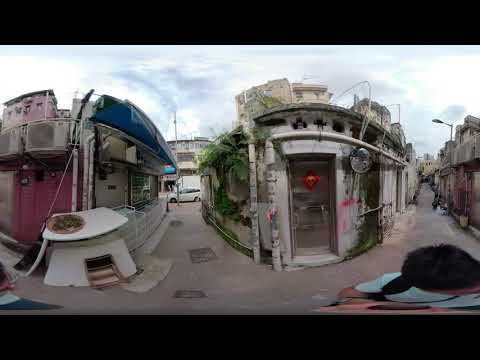This is a skewed photograph of what appears to be a gritty, possibly impoverished, city street. Prominently featuring two main buildings, one on the left and one on the right, both structures exhibit visible signs of decay and neglect, with what might be algae growing up their surfaces. Both buildings have a gray hue, interspersed with faded blue and light purple areas. The left building features a solid pink door, while the right one has an opaque, glass-like door through which the interior is not clearly visible. Running across both buildings are numerous pipes extending towards the rooftops. The image also shows outdoor elements such as air conditioners and lights attached to these buildings.

Supporting structures are partially visible in the background, with one partial building to the right. The street surface appears to be concrete, and in the chaotic composition, there is a table beside the left building and a distorted, almost ghostly image of a person near the bottom right. Additional urban details include sidewalks, parked cars, and more buildings stretching into the background under a partly sunny sky scattered with a few clouds. There are no clear signs identifying any of the businesses, suggesting an indistinguishable and somewhat grim urban setting.